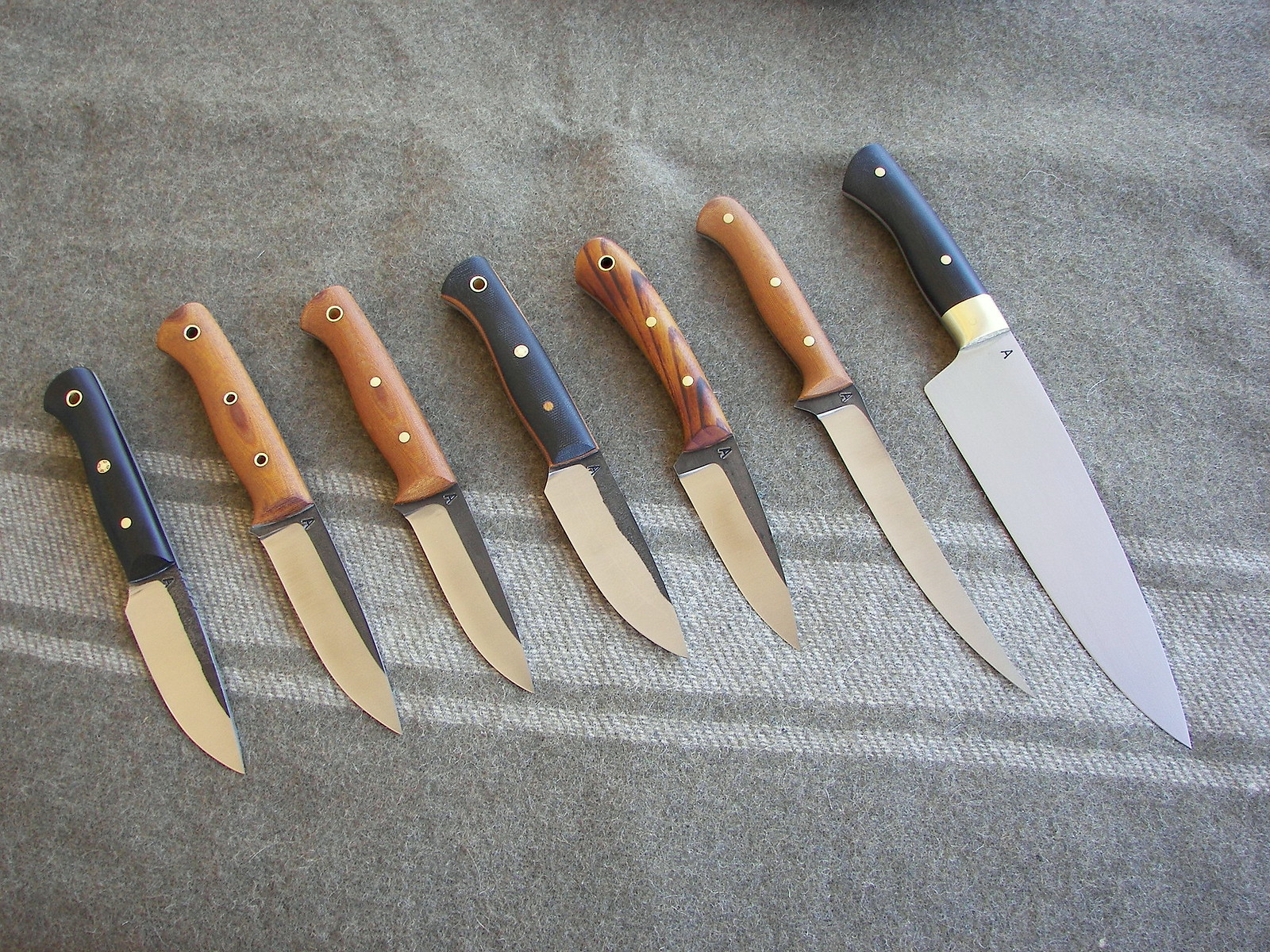In this detailed image, a pristine assortment of seven kitchen knives is meticulously arranged in a row on a textured gray fabric tablecloth with a distinctive pattern: a central white stripe flanked by two gray and white stripes on either side. The arrangement of knives progresses from the largest on the right, a hefty butcher knife with a black handle accented by gold at the juncture, to the smallest on the left, featuring a minimalistic black handle. The knives exhibit a mix of handle colors, predominantly brown and black. One knife showcases an elaborate wood grain handle, contributing to the variety. All the handles are secured by three rivets, except the large butcher knife which has two. The pristine condition of the knives highlights their clean, nearly new appearance against the subtly fuzzy backdrop of the stitched gray cloth.